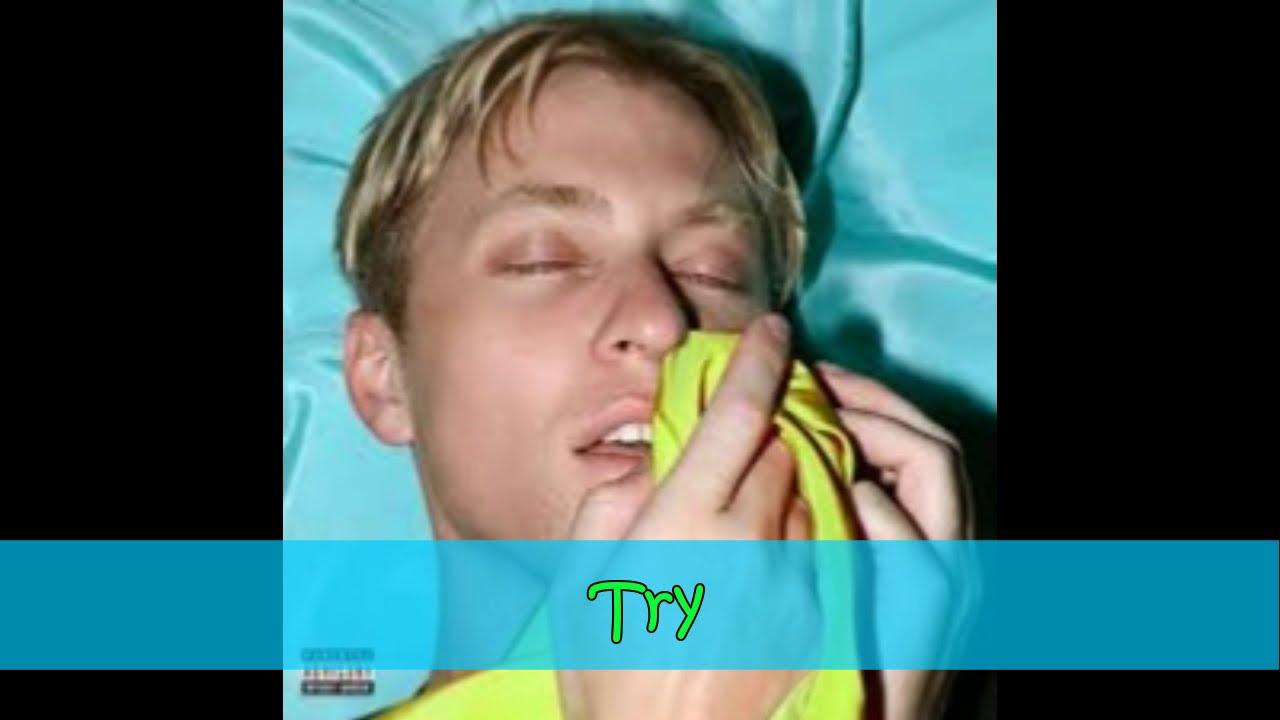This image resembles an album cover featuring a young man with short, blonde hair, resting his head on a blue pillow or sheet. His eyes are closed, and he appears to be either asleep or possibly under the influence of drugs, adding a suspicious aura to the scene. He holds a bright yellow piece of fabric or shirt up to his nose with his hands. The photograph is framed with black bars on either side. At the bottom of the image, a blue streak runs horizontally and contains the word "try" in green lettering. There's a small white label with black text that's too tiny to decipher. Adding to the album cover aesthetic, there's a "Parental Advisory" sticker in the lower right corner. The predominant colors in the image include blue, yellow, blonde, black, and green.